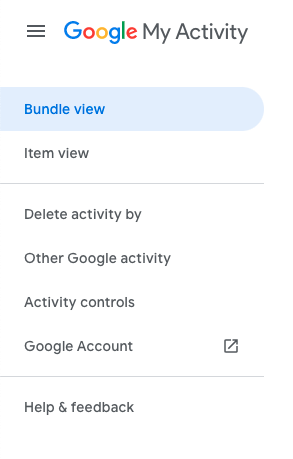This image showcases a Google activity interface, distinguished by its vibrant and colorful design, characteristic of Google’s visual aesthetic. On the left side of this interface, three horizontal lines are displayed, possibly indicating a menu or navigation options. Below these lines, the options are organized in an itinerary format. The first option highlighted in blue is labeled "Bundled View," indicating it is currently selected. Underneath this, another option reads "Item View."

A dividing line runs vertically down the center of the interface, segmenting the remaining sections. Further down, you can see a list of options labeled: "Deleted Activity By," "Other Google Activity," "Activity Controls," and "Google Account." To the right of these labels, there’s a box marked with an upward-pointing arrow, presumably linking to another page or feature. Another dividing line follows this, leading to the final option labeled "Help and Feedback." The background throughout the interface is a clean, uninterrupted white, providing a clear and uncluttered viewing experience.